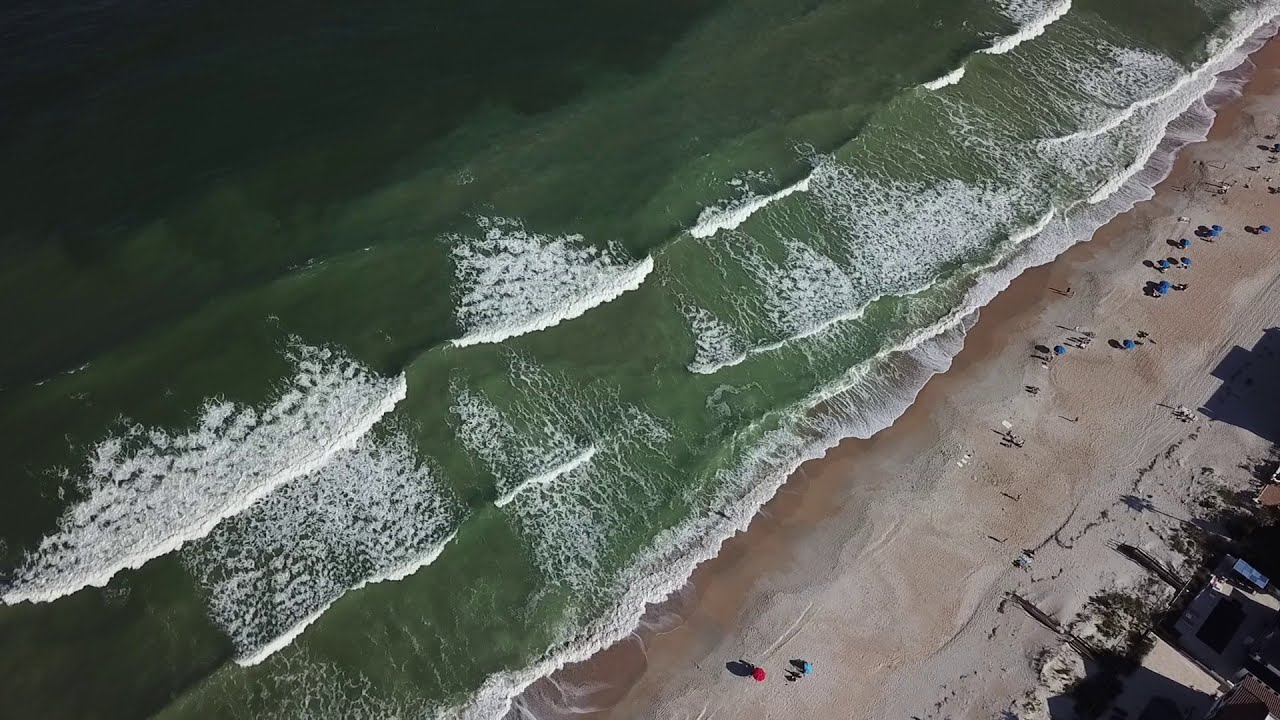This is an aerial drone photograph of a picturesque beach scene viewed directly from above. The image captures the shoreline in vivid detail, with the bottom right and right sides of the photograph showcasing a sandy beach adorned with a few scattered people and two distinct umbrellas, one red and one blue. The majority of beachgoers are clustered in the top right corner, creating a stark contrast with the empty stretch of sand that separates them from the umbrellas.

The sea occupies the entire left side and upper portion of the image, displaying a mesmerizing gradient of water colors that transition from a lighter green near the shore to a deeper, darker green as you move outward. The waves, rolling towards the shore in gentle sets, are topped with white caps, adding a dynamic element to the natural tableau. Near the shoreline, silt and seaweed create a lighter green hue in the water, highlighting the shallows. In the lower right corner, the shadows from nearby buildings begin to creep onto the sand, hinting at the presence of shoreline architecture just outside the frame. The overall scene is serene and uncluttered, captured in the crisp, detailed perspective unique to aerial photography.